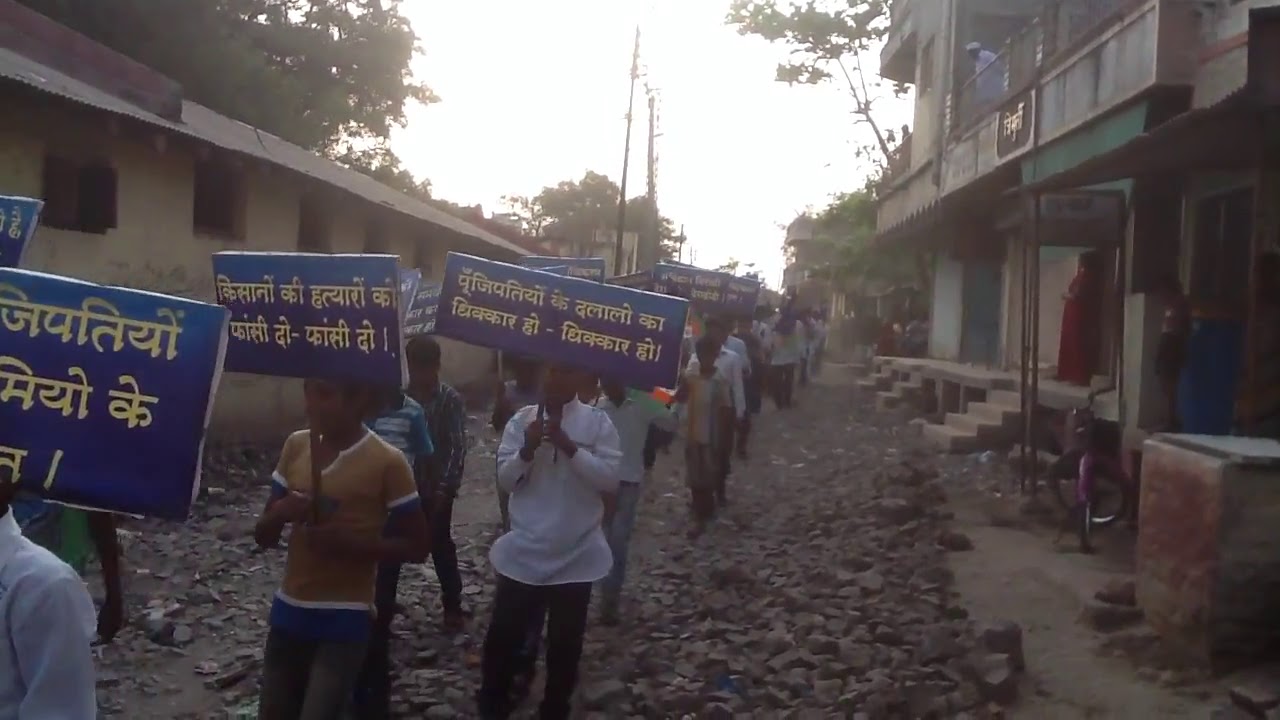The image captures a bustling scene on a hazy day in what appears to be an impoverished village, possibly in India, based on the architecture and street conditions. A long line of people, organized in pairs, marches down a stone-covered side street, holding rectangular blue signs with yellow cursive writing in a non-English language, suggesting a protest. The signs are affixed to poles with a noticeable center spike. The crowd spans hundreds, making their way between two buildings flanking the road. Observing the procession, a man in a white shirt leans over a balcony on the right, while a woman in a red dress stands beneath steps on the left, watching intently. Amid the casual dress of the marchers, one man is identifiable in a white long-sleeve shirt and dark pants, and another in a yellow short-sleeve shirt. A purple bicycle rests on the right side of the rugged, rubble-strewn street, adding to the scene’s vivid detail.